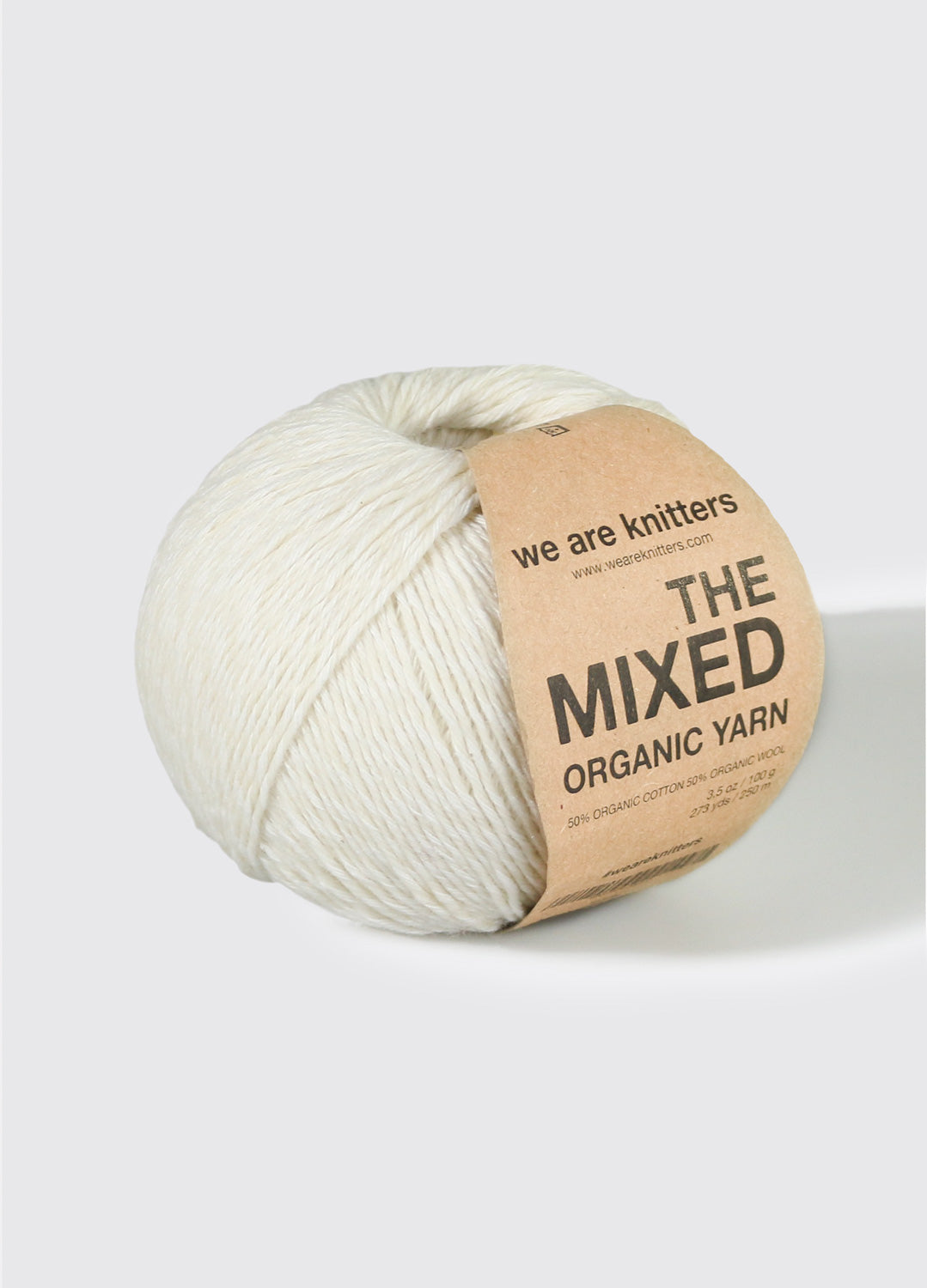This detailed photograph depicts a brand new ball of yarn resting on a completely white table with a matching white background, contributing to a minimalistic and clean aesthetic. The ball is neatly wound in a cross-folded manner, revealing layers beneath the surface layer, and has a characteristic squat, round shape with a prominent central hole, making it easy to grab. The yarn itself is white, though it appears slightly different in tone compared to the pure white background.

A brown cardboard label wraps around the ball, lending it a rustic, eco-friendly look reminiscent of recycled packaging. The label prominently features the brand name "We Are Knitters" in black text, accompanied by the website "www.weareknitters.com." Beneath this, larger text states "The Mixed Organic Yarn" along with details indicating a blend of 50% organic cotton and 50% organic wool, and the weight of 3.5 ounces (100 grams). Additional smaller text and a barcode are also present, although these details are less readable.

Light sources seem to be off to the left, as evidenced by the shadow cast to the right of the yarn. This pristine and orderly presentation suggests the yarn is in its original packaging, untouched and ready for use in knitting or crochet projects.